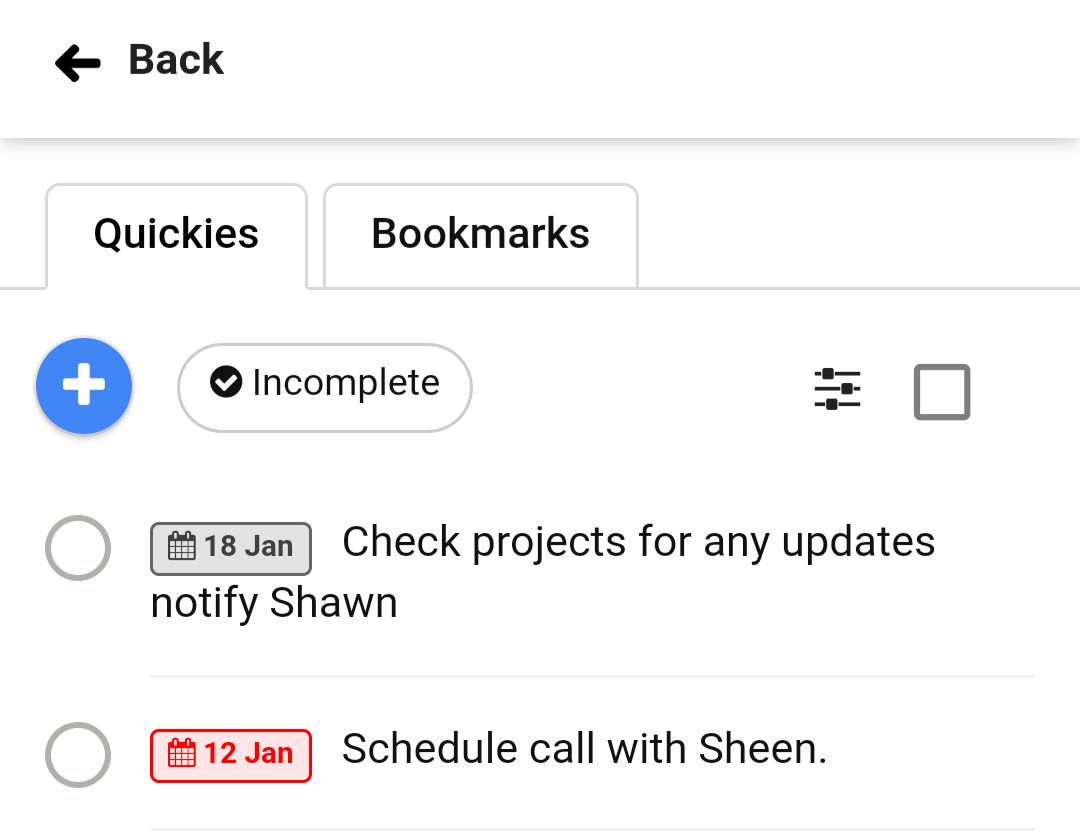In the top left corner of the interface, there is a bold, rounded black arrow pointing to the left with the word "Back" in black, bold text, capitalized. This section is separated by a divider line with a light gray shadow effect beneath it. Below, there are two tabs labeled "Quickies" and "Bookmarks," with "Quickies" currently selected.

Directly below the selected tab, there is a blue-filled bubble containing a white, bold plus sign. To its right, an oval-shaped icon with a white background and light gray border houses a small black circle in the left side, featuring a white check mark. To the right of this icon, the word "Incomplete" is written in black.

Farther to the right, there are three adjustable menu lines. Each line has a square alternately positioned on the left or right. To the right of these lines, there is a light gray bordered box that is not checked. Below this, in the next line, an unselected radio button with a light gray outline appears, followed by a small rectangular icon with a rounded gray border. Inside this icon, there is a gray calendar icon next to the text "18 JAN" in gray. 

To the right of this text, it says in black, "Check progress on projects for any updates. Notify Sean."

Underneath, on the left, another unselected radio button with a gray border is visible. To the right, a rectangular icon appears with a light red background, dark red border, and dark red calendar icon, along with the text "12 Jan" in bold dark red. To the right of this, in black text, it says, "Schedule call with Sheen."